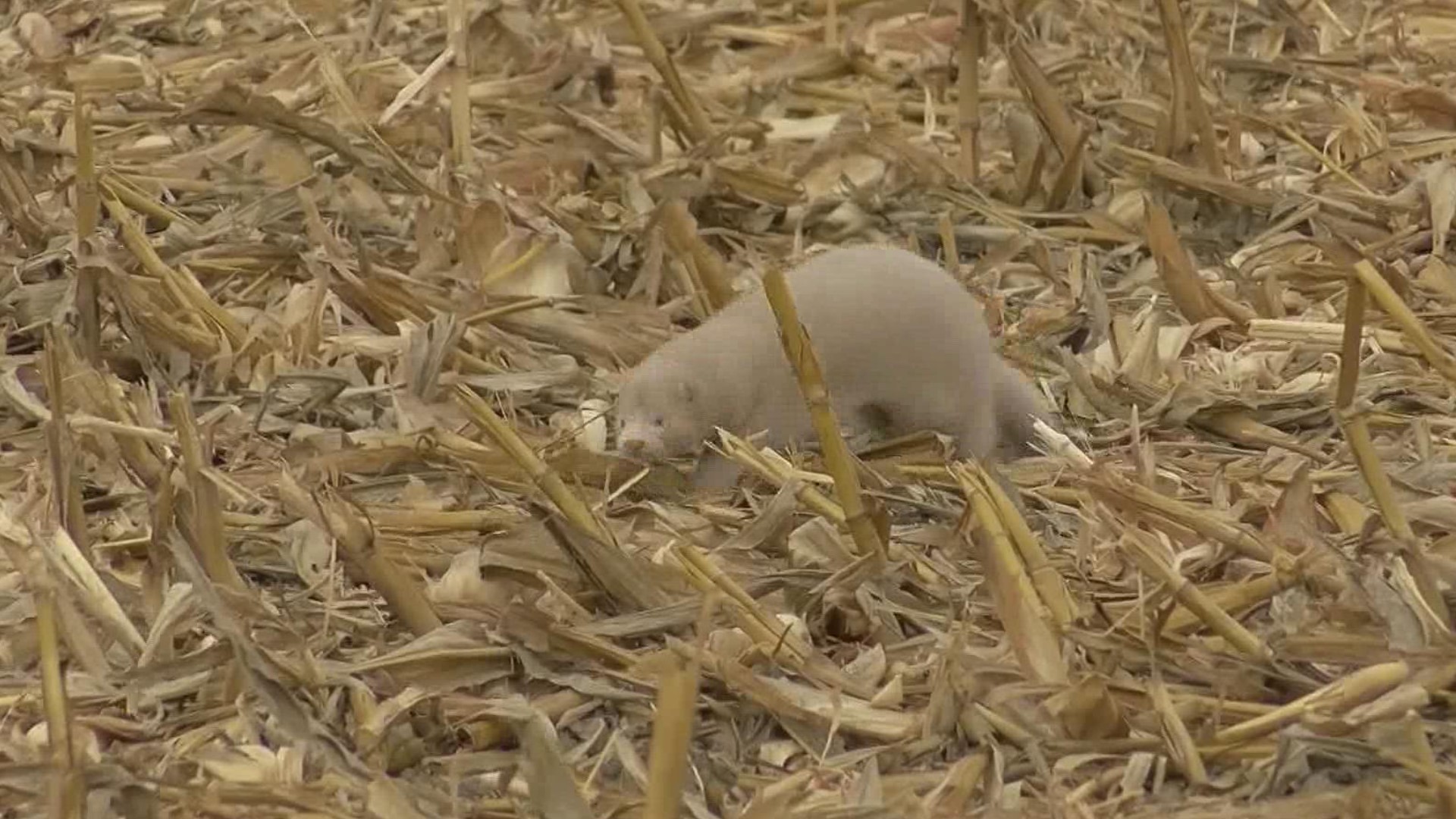The photograph captures a small, light-colored mammal situated in a field of dry, brown vegetation. The animal, which is all white or light beige with tiny eyes, a grey nose, and small ears, resembles a bear but is significantly smaller, more akin to the size of a gerbil or hamster. The setting, likely in the summertime, appears to be an area with dried hay or cut bamboo, evidenced by the numerous plant pieces scattered across the ground, looking either cut or severely damaged. The animal is positioned somewhat centrally in the frame, and despite the distance of about 10 to 20 feet, its features remain clearly visible. The dry brush around it lacks context clues to provide a definitive sense of scale.